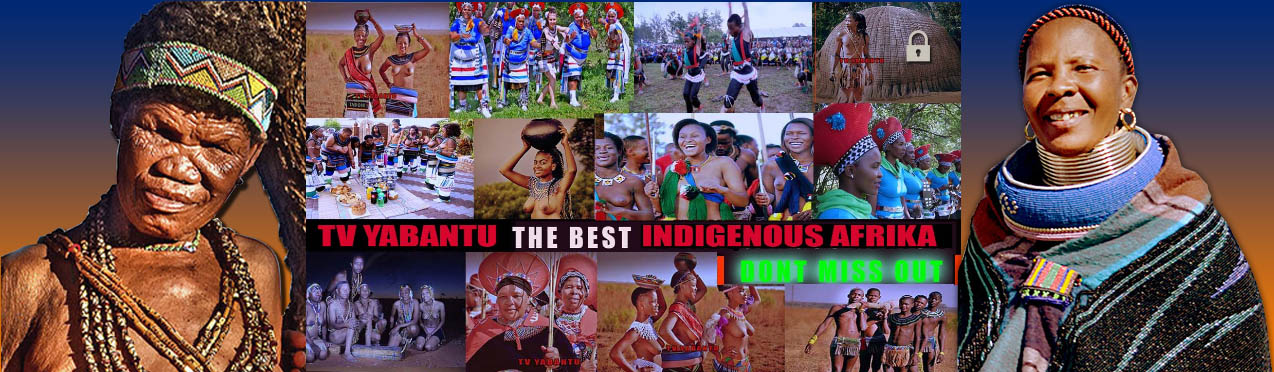A vibrant and detailed collage image features a series of photographs set against a blended dark blue-to-orange background. This horizontal landscape composition prominently displays two tribal elders on either side, both dressed in traditional attire. On the left, an older woman, with hair tied up and adorned with a geometric-shaped headband, wears minimal clothing and a plethora of beaded necklaces. The right side features another woman wearing a headband, silver hoop earrings, a tight silver collar, and a larger blue collar, draped in a blanket and smiling at the camera. The central section is a rich mosaic of various scenes showcasing African men and women immersed in traditional ceremonies and daily activities. Many women in these images are topless, and some balance objects on their heads, while others wear more elaborate traditional outfits. Three-quarters down from the top, a black background displays the text "TV Yabantu" in red, "The Best" in white, and "Indigenous Africa" in red, with the phrase "Don't Miss Out" in green text on the right side.